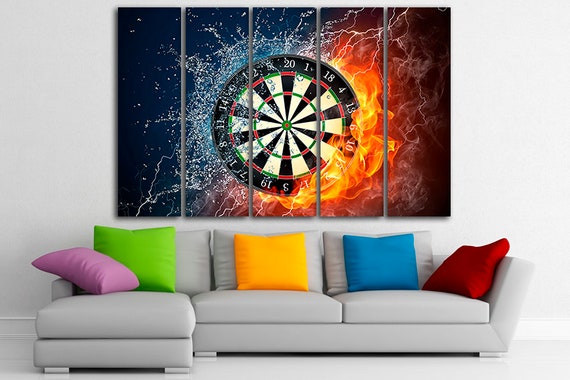The living room features a light gray leather sofa, accented with colorful throw pillows arranged in a specific order: from left to right, there’s a pink, green, orange, blue, and red pillow. A smaller purple pillow is placed sideways on the arm of the couch. The wall behind the sofa is light gray with a white baseboard, and the flooring appears to be light gray tile.

Above the sofa hangs a large, horizontally-aligned rectangular painting divided into five vertical sections. This artwork depicts a dynamic scene centered on a dartboard encased in contrasting elements: the left side is engulfed in water with shades of black and blue, while the right side is ablaze with red and orange flames. Lightning bolts strike across the dartboard, adding an electrifying effect. The detailed composition of the painting enhances the modern and eclectic vibe of the room.